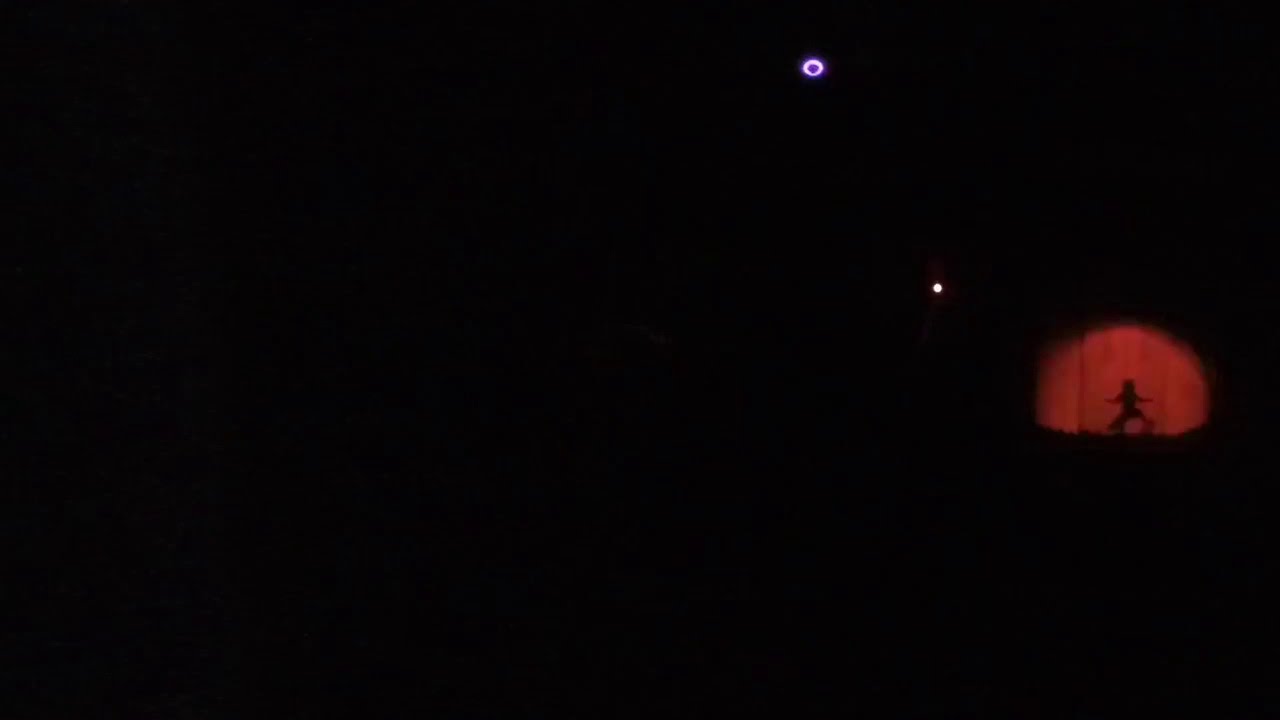The image captures a nighttime stage performance shrouded in darkness, with a majority of the composition being pitch black. At the center-right portion of the image, taking up about a tenth of the total space, a red spotlight illuminates a maroon curtain, casting the shadow of a dancer in a squat position with arms extended. This silhouette of a woman is a striking feature, making it appear as though she is performing at a raised level on the stage. Above the stage, two small lights are visible — a circular light and a white dot, contributing minimal illumination. The rest of the room is enveloped in darkness, obscuring any details of the audience or surroundings.